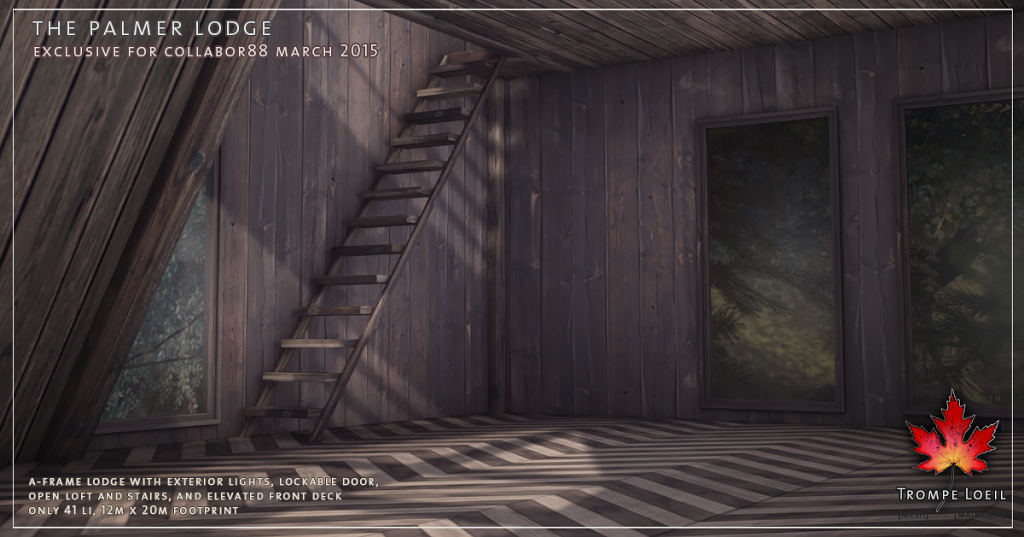The image features an advertisement for a 3D model of the Palmer Lodge, specifically designed for the Collab88 event in March 2015. It showcases the interior of a wooden cabin, complete with an open, airy loft accessible by a wooden staircase on the left side. The cabin includes three windows: one triangular window on the left and two tall, rectangular windows on the right, offering a view of trees outside. The floor is adorned with a zigzag patterned carpet in dark gray and lighter white stripes. The image is framed by a thin white border, with detailed text at the top left stating, “The Palmer Lodge, exclusive for Collab88 March 2015,” and additional descriptive text at the bottom left specifying features such as exterior lights, a lockable door, an open loft, stairs, and an elevated front deck. The listed footprint of the lodge is 12 meters by 20 meters. In the bottom right corner, there is a red maple leaf with tints of gold and orange, underneath which is the text “Trompe Loeil.”